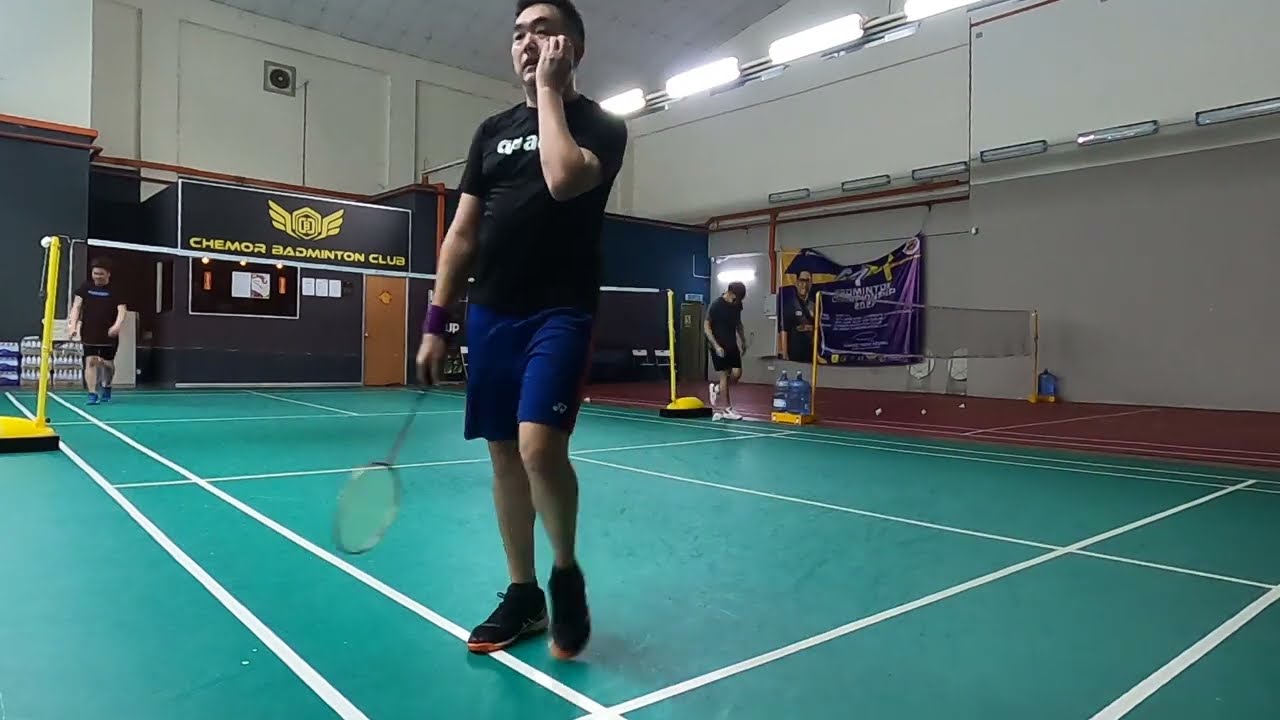In this detailed image, a middle-aged Asian man is standing near the corner of a green and white-lined racquetball court, which is part of the Chemore Badminton Club, as indicated by a black and yellow banner visible in the background. He is dressed in a black t-shirt, blue shorts, and black shoes, holding a badminton racquet in his right hand while his left hand touches his cheek. Positioned across the net, which features yellow railings and a white net, is his opponent, similarly attired in a black shirt, black pants, and blue shoes. The gymnasium has white walls and a neighboring red court adjacent to the green one.